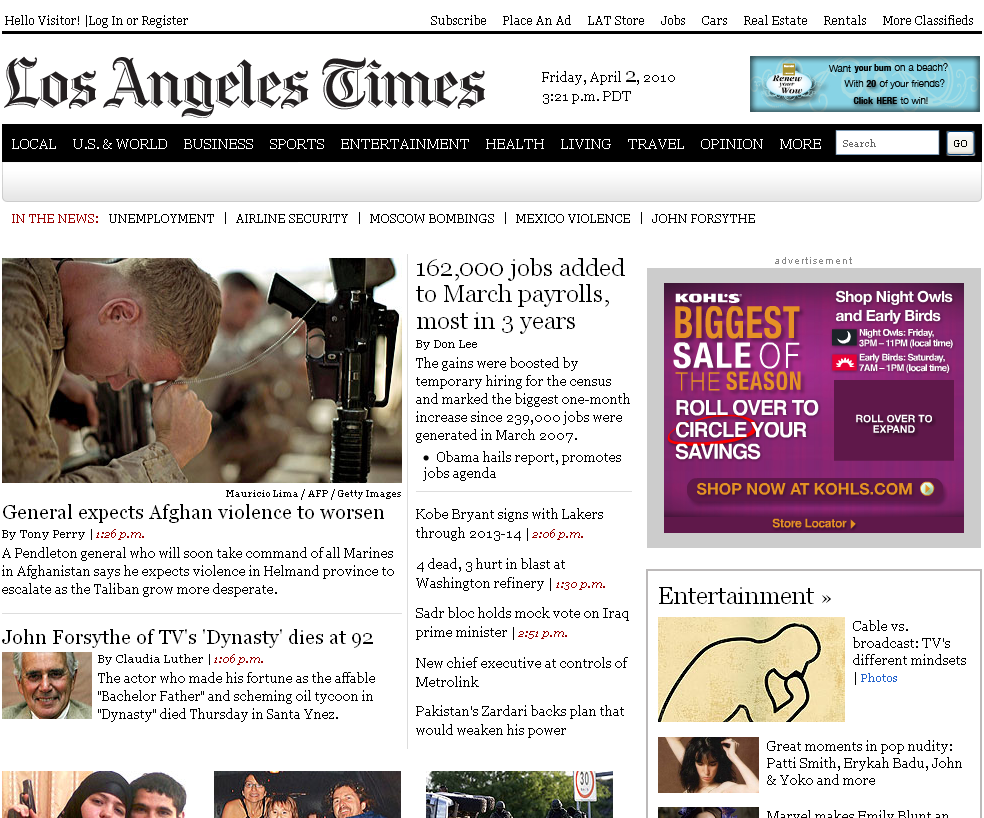**Caption:**

A detailed screenshot of the Los Angeles Times website, dated Friday, April 2nd, 2010 at 3:21 p.m. Pacific Daylight Time. The website's top navigation bar includes options such as "Hello Visitor, Log In or Register," "Subscribe," "Place an Ad," "LAT Store," "Jobs," "Cars," "Real Estate," "Rentals," and more classified sections. Additionally, there's a promotional button with the text "Want Your Bomb on a Beach with 20 of Your Friends? Click Here to Win. Renew Your Wow."

The main navigation tabs are: Local, U.S. & World, Business, Sports, Entertainment, Health, Living, Travel, Opinion, and More. A search button is also available for finding specific content.

Underneath the main menu, there's a section labeled "In the News," featuring tabs for hot topics including Unemployment, Airline Security, Moscow Bombings, Mexico Violence, and John Forsythe. Highlighted articles include:

1. "General Expects Afghan Violence to Worsen," featuring an image of a dejected man with his head down and weapon in hand.
2. "John Forsythe of TV's Dynasty Dies at 92"
3. "162,000 Jobs Added to March Payrolls, Most in Three Years"

Additionally, a Kohl’s advertisement promoting "The Biggest Sale of the Season" is visible, encouraging users to "Roll Over to Circle Your Savings, Shop Now at Kohls.com." Other highlighted content includes articles on the differing mindsets between cable and broadcast TV, among various other news stories.